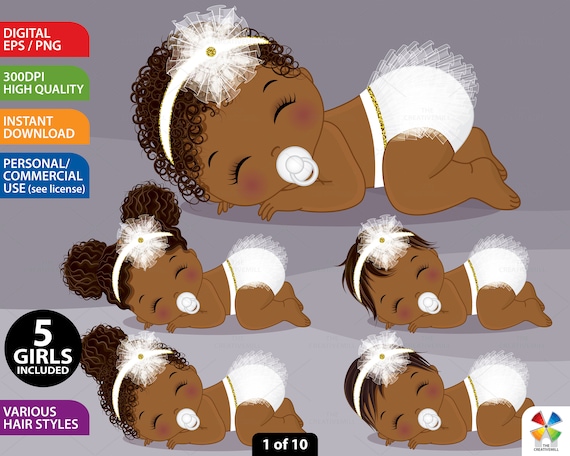This image presents a whimsical scene featuring five African-American baby girls drawn in a cartoon-like style. Each baby is positioned while lying on their belly, all dressed identically in white, lacy diapers and donning matching white headbands adorned with lacy star-shaped decorations. They are all sucking on white pacifiers and their heads are uniformly turned to the left. The distinguishing feature among these babies is their diverse hairstyles: the largest baby at the top flaunts very curly hair, while the two babies directly below her display pixie cuts; the last two babies, positioned at the bottom, showcase a braid bun and double bun braid hairstyles, respectively.

The background transitions from medium gray at the top to a lighter gray at the bottom. Positioned to the left of the largest baby at the top, various sections of text are displayed on colored backgrounds, potentially indicating an advertisement for a digital template. In white letters on a red background, it reads "Digital EPS/PNG"; below on a green background, "300 DPI High Quality"; further down on an orange background, it states "Instant Download"; followed by a blue section reading "Personal/Commercial Use"; and finally, a black circle in the lower left corner declares "Five Girls Included," with a purple section beneath that detailing "Various Hairstyles." The baby's delicate features are subtly enhanced, with a touch of rouge on their cheeks and highlighted eyelashes, adding to the charm of the illustration.